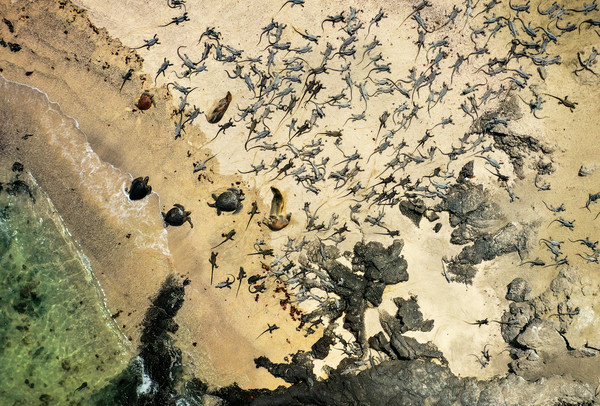The image is a fascinating aerial photograph capturing a bustling beach scene, quite possibly in the Caribbean or a similar coastal region. Dominating the scene are four adult sea turtles situated close to the green-tinged water at the lower left-hand corner. Scattered across the rest of the sandy beach are hundreds of smaller creatures, which appear to be baby sea turtles; although, their long bodies and tails lend them a resemblance to lizards or geckos. The smaller turtles, sprawling from the middle of the image towards the top right-hand corner, create a striking visual. Among the mix, there are some indistinct shapes that might be other animals, adding an element of mystery. The beach itself alternates between wet and dry sand, interspersed with brown rocks and possibly caves, providing a textured backdrop to this extraordinary natural spectacle.